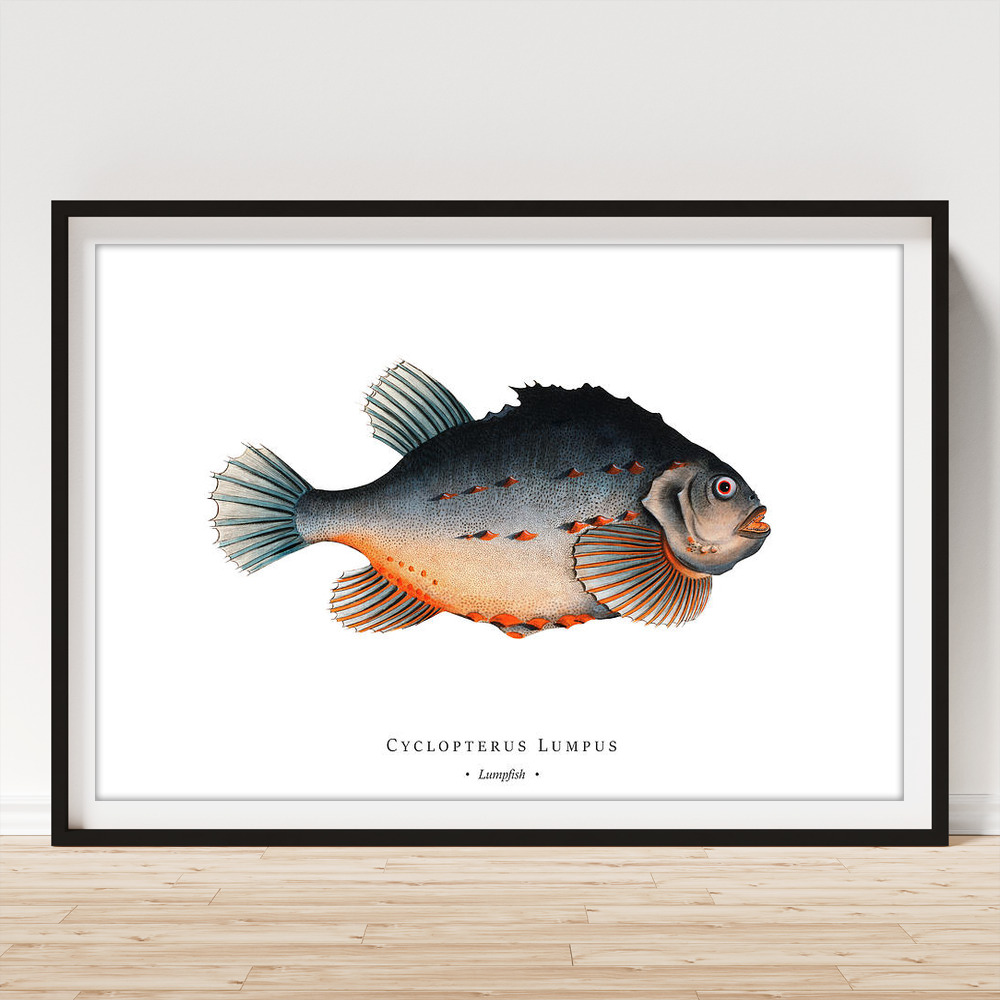This photograph captures a large framed art piece, possibly measuring around six by five feet, leaning horizontally against a pristine white wall. The floor beneath it is a light beige wood, contributing to the room’s overall light and airy ambiance. The artwork itself is a detailed illustration of a fish, prominently labeled at the bottom as "Cyclopterus lumpus" in bold text, with "Lumpfish" written beneath in smaller font. The fish’s body is a blend of dark blue upper parts and lighter tan underparts, accented with orange highlights on its stomach, some fins, and parts of its mouth. Its vivid red eyes gaze directly at the viewer, creating a captivating contrast against its side profile. The illustration features intricate details: light blue and dark blue outlined fins, an orange outline on the lower fin below the gill, and additional orange spikes, making the bottom half of the fish more orange-leaning. The entire background of the artwork is white, and it is encased in a black-rimmed frame with a light gray inner border about an inch wide, enhancing the overall presentation.